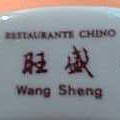The image is a very small, slightly grainy, color close-up photograph of what appears to be the underside of a piece of porcelain, possibly a plate or cup, due to the visible curved and rounded edge. The background of the image features a thin horizontal strip of coral or reddish-orange color at the top. The main object is white with a bluish tint, and prominently displays black capitalized lettering that reads "RESTAURANTE CHINO." Beneath this text, there are two Chinese characters, with the left character labeled "WANG" and the right character labeled "SHENG." The lower part of the image is marginally darker than the top, enhancing the appearance of a maker's mark or stamp on the porcelain surface.